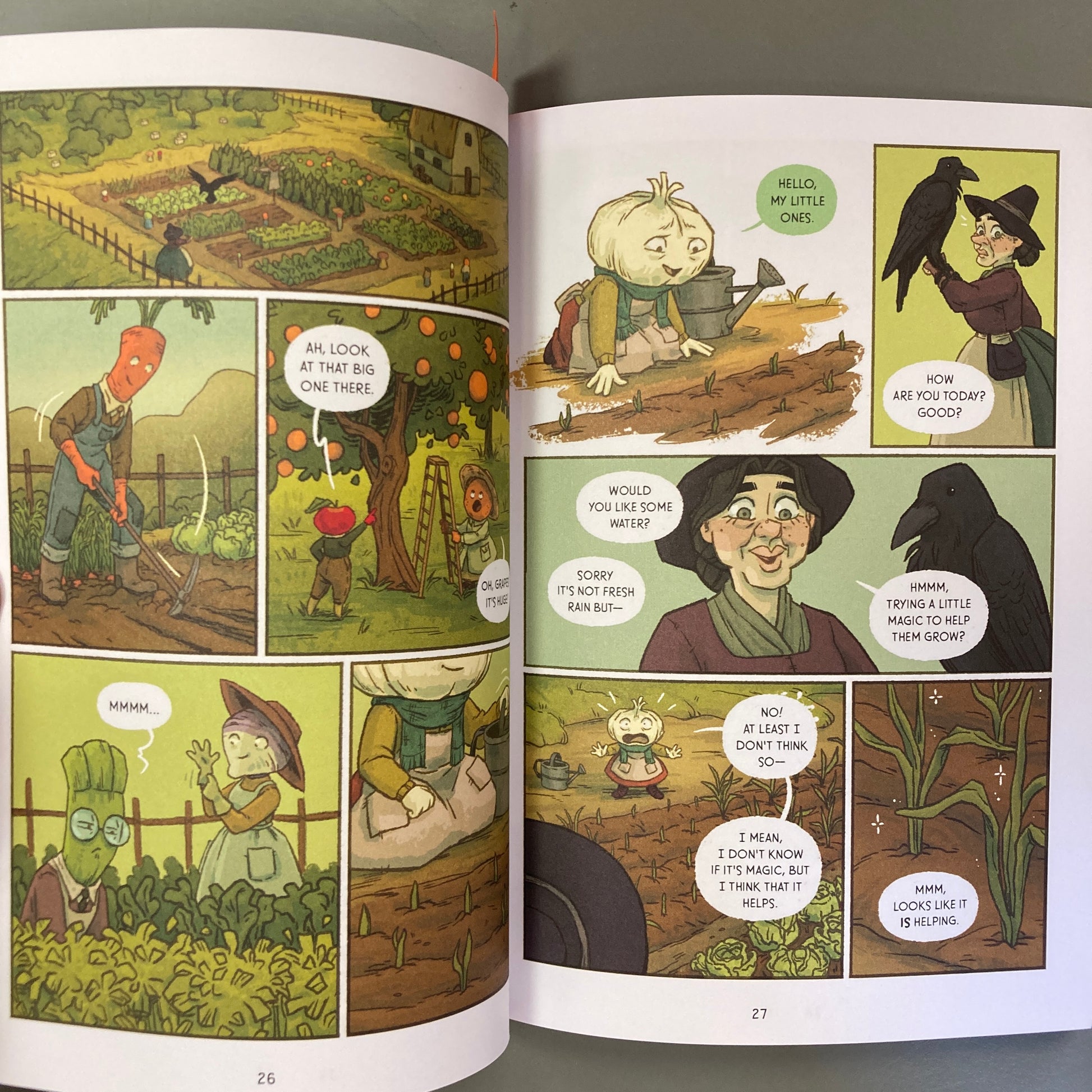The photograph captures a comic book opened to pages 26 and 27, laid flat on a gray surface, likely a table or desk. The comic features whimsical, anthropomorphic vegetable characters in a farm setting. On the left page, the first panel showcases an aerial view of a farm with a carrot-headed character wearing overalls and using a pickaxe in the soil. Below this panel, an asparagus and turnip-headed characters are looking at crops. On the right page, a female human farmer, dressed in typical farmer’s attire, greets the vegetable characters with “Hello, my little ones.” A childlike figure with an apple head and wearing pants points towards an orange tree, exclaiming, “Ah, look at that big one there.”